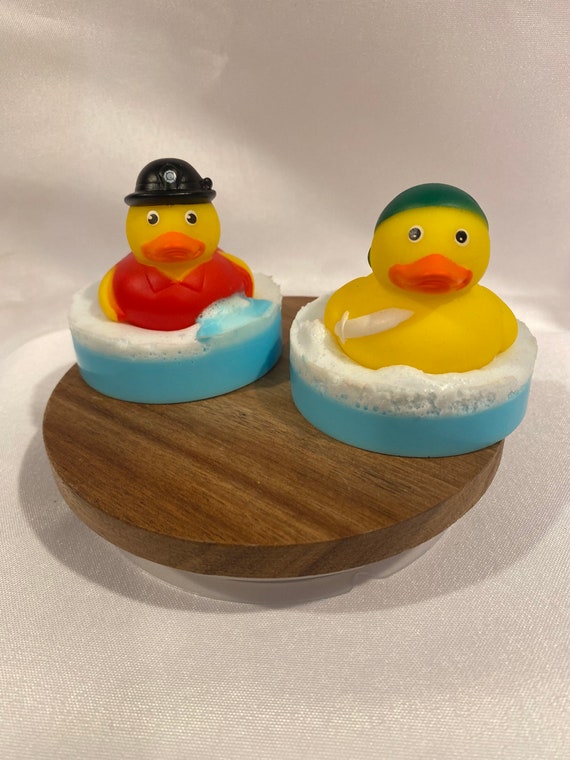This is a close-up color photograph depicting two floating rubber toy ducks on a wood grain turntable, set against a professionally arranged wavy off-white background within a photo booth. Both ducks are perched on circular green pods that simulate water with artificial suds and soap. The duck on the right wears a backward green baseball cap and has an orange body. Its pod features blue water at the base with white foam on top. This duck also has an accessory resembling a white sword, giving it a pirate-like appearance. The duck on the left sports a red vest and red bow tie, topped with a bowler-type cap (described as black helmet in one instance). This duck’s pod setup mirrors the one on the right, complete with soap suds. Both ducks have orange beaks and share the same yellow rubber material, creating a whimsical, well-composed scene designed to highlight the detailed miniature bath-time setting.